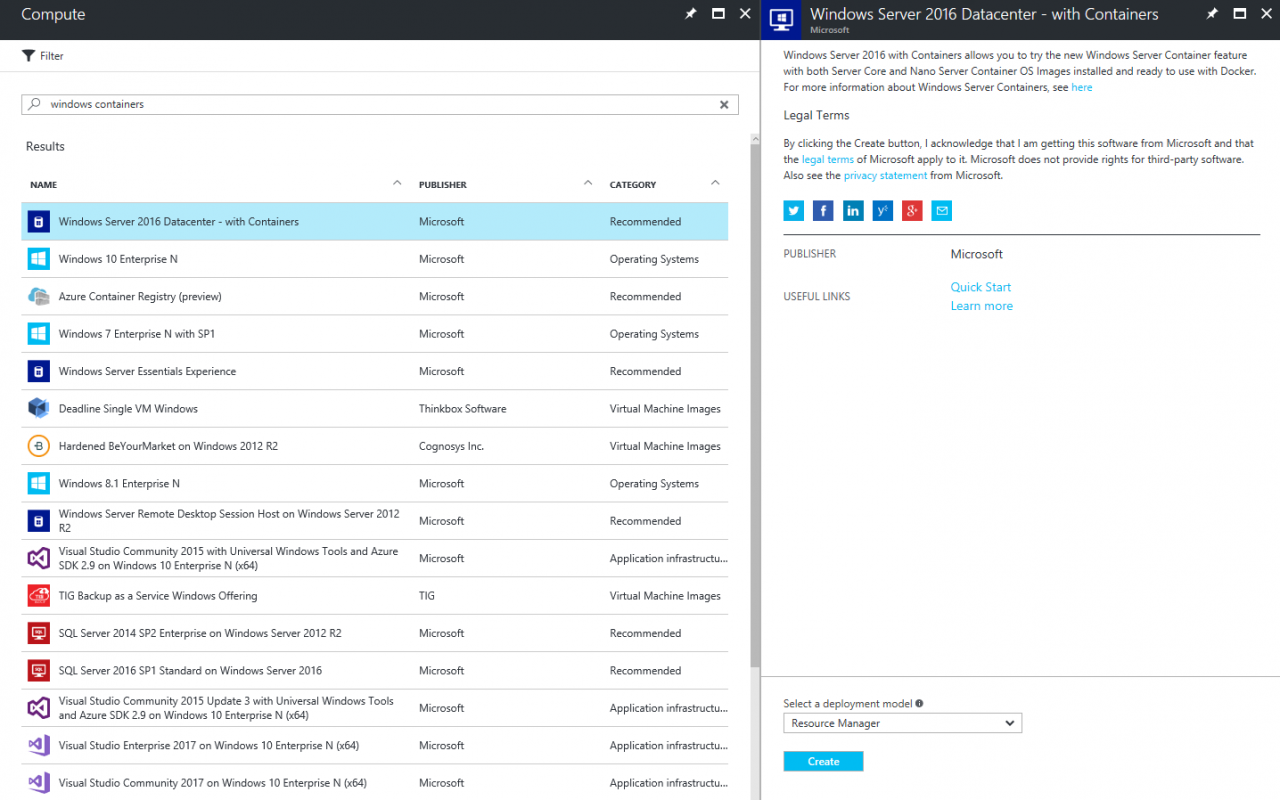The image captures a detailed interface presumably of a software or cloud management platform. At the top of the interface, there's a horizontal search bar displaying the text "Complete Compute." Directly below, the window is split into two distinct sections:

**Left Section:**
- A search bar at the top with the phrase "Windows containers" typed in. The search bar features a magnifying glass icon to the left and an "X" button to the right.
- Beneath the search bar, a list of Windows programs is displayed in tabular form. The columns are labeled "Name," "File User," and "Categories."
- The list includes various Windows products such as "Windows Server 2016 Datacenter," "Windows 10 Enterprise," "Windows 7 Enterprise," "Visual Studio," "SQL Servers," and more, each accompanied by details about their publisher and category.

**Right Section:**
- The top of this section has a black banner with the text "Windows Server 2016 Datacenter with Containers."
- Below the banner, there is small, hard-to-read text that includes information such as the publisher ("Microsoft"), links for "Useful links," "Quick start," and "Learn more."
- At the bottom of this section, the term "Resource Manager" is visible next to a prominent blue button labeled "Create."

The interface appears to be expertly designed for navigating and managing various Windows programs and servers, offering users a structured and comprehensive tool.